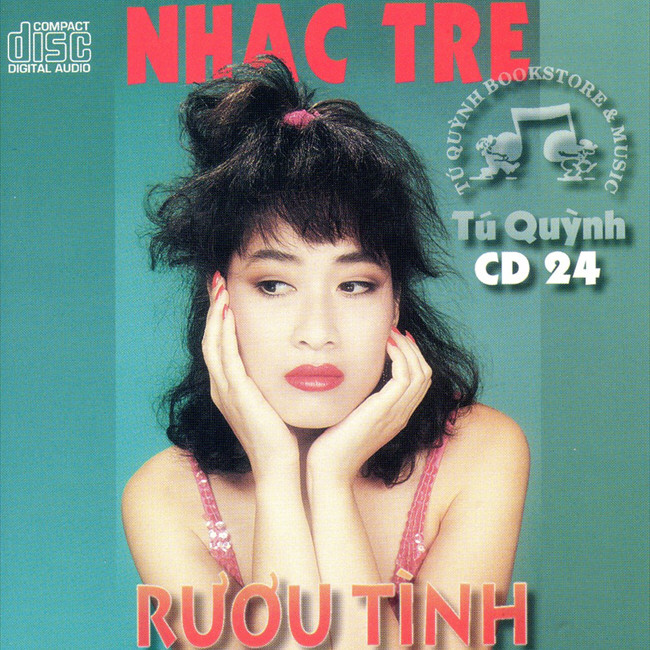The image is an advertisement for a CD, possibly from Vietnam. At the center of the image is a young Asian woman with long, flowing black hair styled into a partial ponytail, gazing off to the side with her chin resting on her hands. She is dressed in a delicate pink sequin tank top and wears subtle eyeshadow, eyeliner, and red lipstick. The background is a bluish-green color, which contrasts with the bold, red text on the image. 

At the top of the image, "N-H-A-C-T-R-E" is written in prominent red letters. Below the woman's image, another line of red text reads "R-U-O-U-T-I-N-H." 

Additionally, in the upper left corner, the logo "Compact Disc Digital Audio" is displayed in white, while in the top right corner, the text "T-U-Q-U-Y-N-H Bookstore and Music" and "CD 24" are inscribed. The overall design indicates that this is a CD cover for a Vietnamese singer named Thu Quynh.